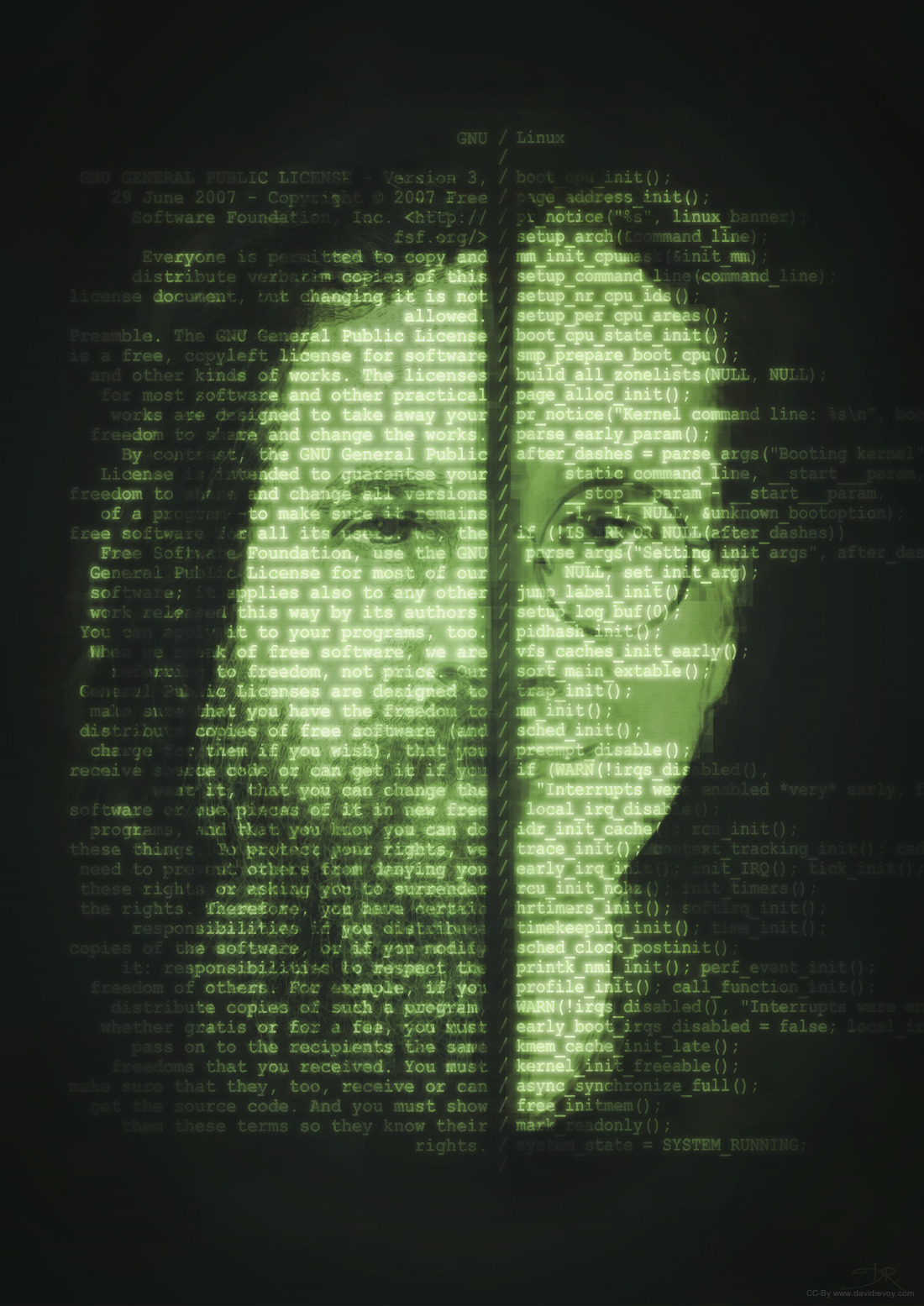The image displays a digital photo of a screen, possibly a screenshot or a printout. This screen showcases an artistic rendering of a human face, executed entirely through strategically placed text. The face, which appears to be male with dark hair, is detailed using a clever interplay of light and dark shadows created by the text. The facial features, including the eyes, eyebrows, nostrils, a line for the mouth, and the neck, are clearly discernible. 

Embedded within the face are lines of text featuring phrases such as "general public license," "boot CPU state," "licenses build all zone lists," "another line and change the works," "early param," "foundation use the GNU args setting," "that you have the freedom," "them if you wish," "or can get it if you," "that you can change interrupts," and "copies of such a program." These textual elements suggest the inclusion of technical and open-source software terminology, adding layers of depth and meaning to the artistic representation.